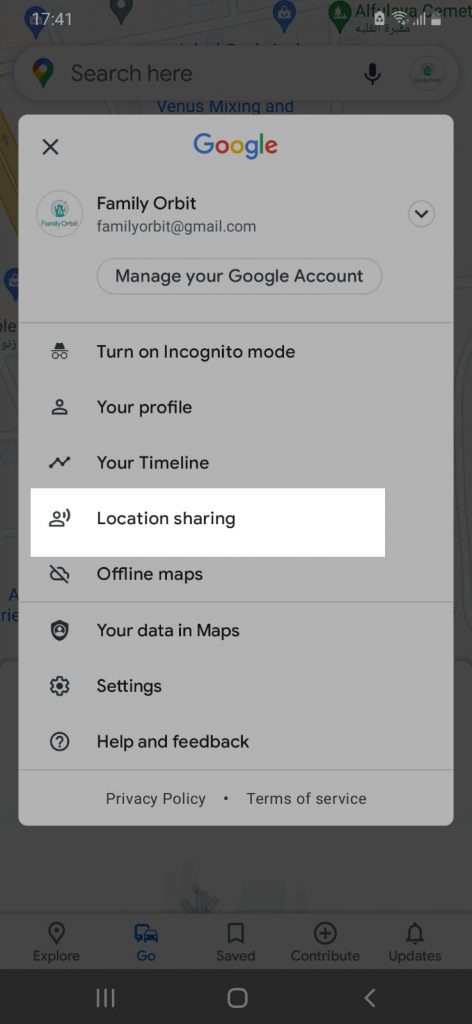The image showcases a Google pop-up on a smartphone screen. At the top of the screen, the status bar displays the time as 17:41, a Wi-Fi connection icon, a signal strength icon, and a battery icon indicating about 50% charge. The Google pop-up features a gray background with the word "Google" prominently at the top and an 'X' icon in the top left corner for closing the pop-up.

Below the Google header, the email address "familyorbit@gmail.com" is shown, followed by the option to "Manage your Google Account." A list of categories is presented in black text, starting with "Turn on incognito mode," "Your profile," and "Your timeline." The option "Location sharing" is highlighted with a white rectangle. Following this are "Offline maps," "Your data in Maps," "Settings," "Help & feedback," and finally, smaller text at the bottom indicating "Privacy policy" on the left and "Terms of service" on the right.

The background of the pop-up has a holographic effect at the top and bottom, revealing that the underlying screen is a map from Google Maps. At the very bottom of the entire image is a black navigation bar featuring three icons: on the left, three vertical lines; in the center, a circle; and on the right, an arrow pointing left.